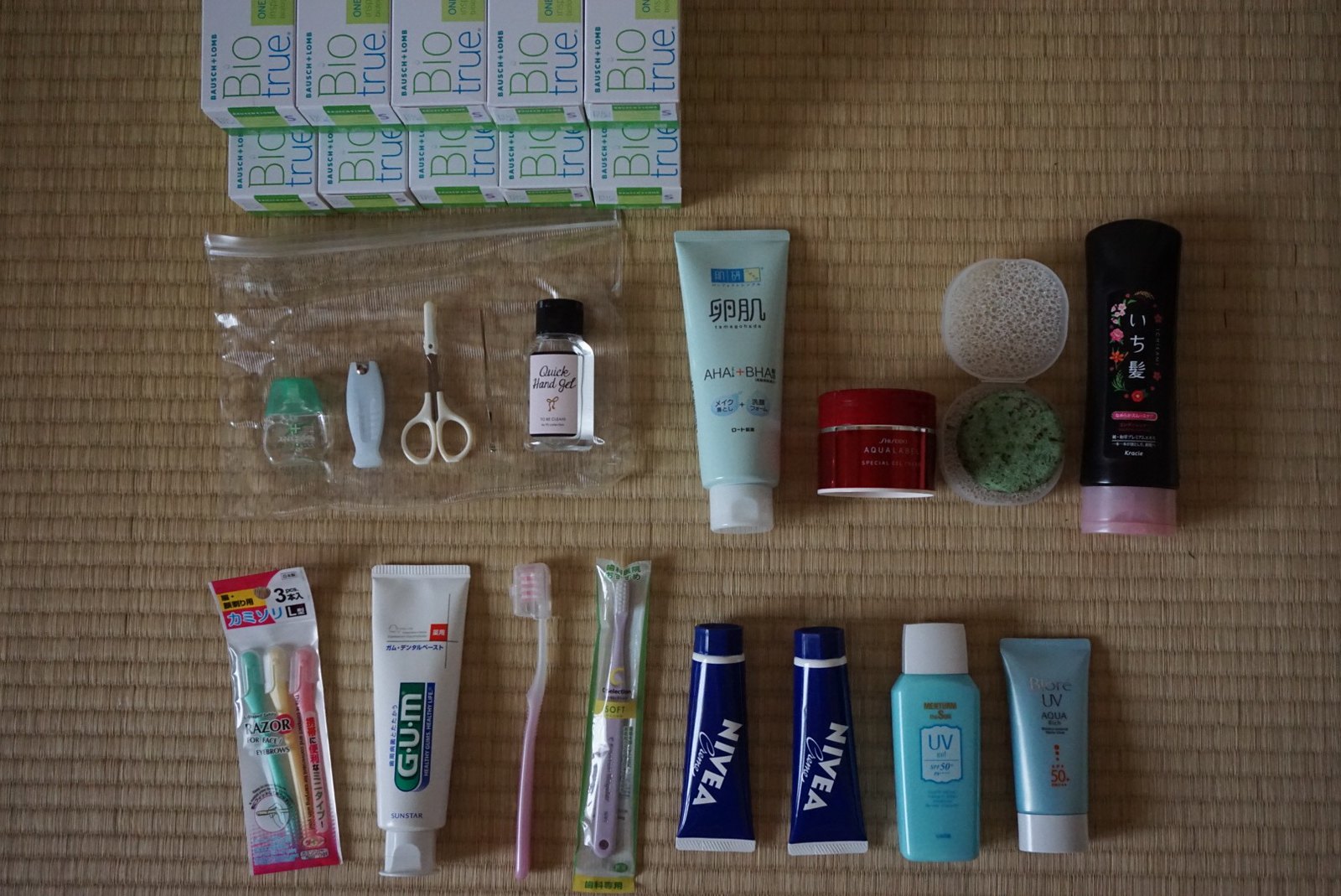This photograph showcases a meticulously arranged collection of hygiene supplies, displayed on a tightly coiled mat with a bamboo-like beige and brown pattern. Natural light from a window on the left illuminates the scene, leaving the right side slightly shadowed, suggesting that a flash might have enhanced the clarity.

At the top left corner of the image, ten white boxes with blue writing and green detailing are stacked in two rows. The boxes are labeled "Bio True" and are positioned in a staggered formation to reveal all product labels clearly. Below these boxes is a clear Ziploc-style bag containing various items: a small clear bottle with a pink label and black lid, a pair of pale yellow nail scissors, white nail clippers, and a green and clear object of undetermined use.

To the right of the bag, there is a sequence of various containers. First, a pale blue tube with a blue and white logo and black scroll font. Next to it sits a round tub with a metallic red label and matching red lid, followed by what appear to be sponges. Adjacent to the sponges is a black bottle-style container with a red lid, featuring a multi-colored label.

The bottom row features additional hygiene items. Starting from the left, there are three toothbrushes or flossing tools in plastic packaging, followed by a white tube labeled "GUM" against a blue background. Next in line is a pale pink toothbrush with bristles facing left. Another brush, encased in a plastic holder, sits beside a duo of Nivea cream tubes placed upside down with their caps facing up. The row concludes with a baby blue bottle and matching blue tube, both with white lids, with the bottle indicating "UV" suggesting they might be sunblock products.